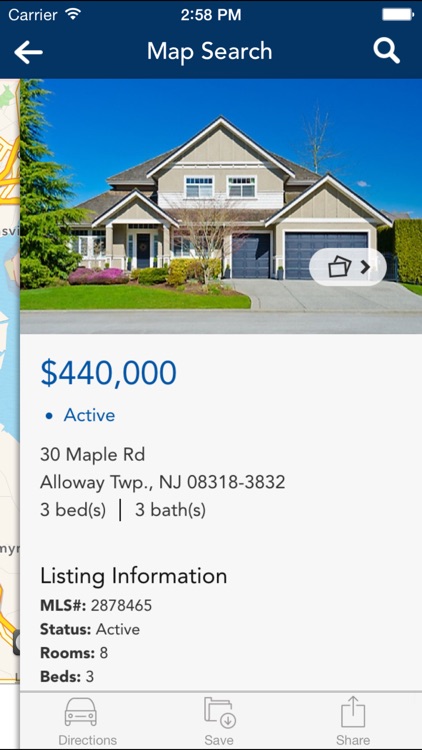Screenshot of a real estate app showcasing a detailed listing for a property located at 30 Maple Road, Aloe, New Jersey. The property is marked as "active" and is listed for $440,000. The home resides within a suburban neighborhood and features two stories with beige-colored walls and distinct blue garage doors, including one large and one smaller door. It includes a well-maintained lawn adorned with a massive pine tree to the left and nicely trimmed bushes, one exhibiting dim purple leaves. The backyard has an additional tree without leaves. The listing details specify that the house includes eight rooms in total, three bedrooms, and three bathrooms. The MLS listing number is also provided. The sky in the image is crystal clear, enhancing the appeal of this charming, recently-built home.